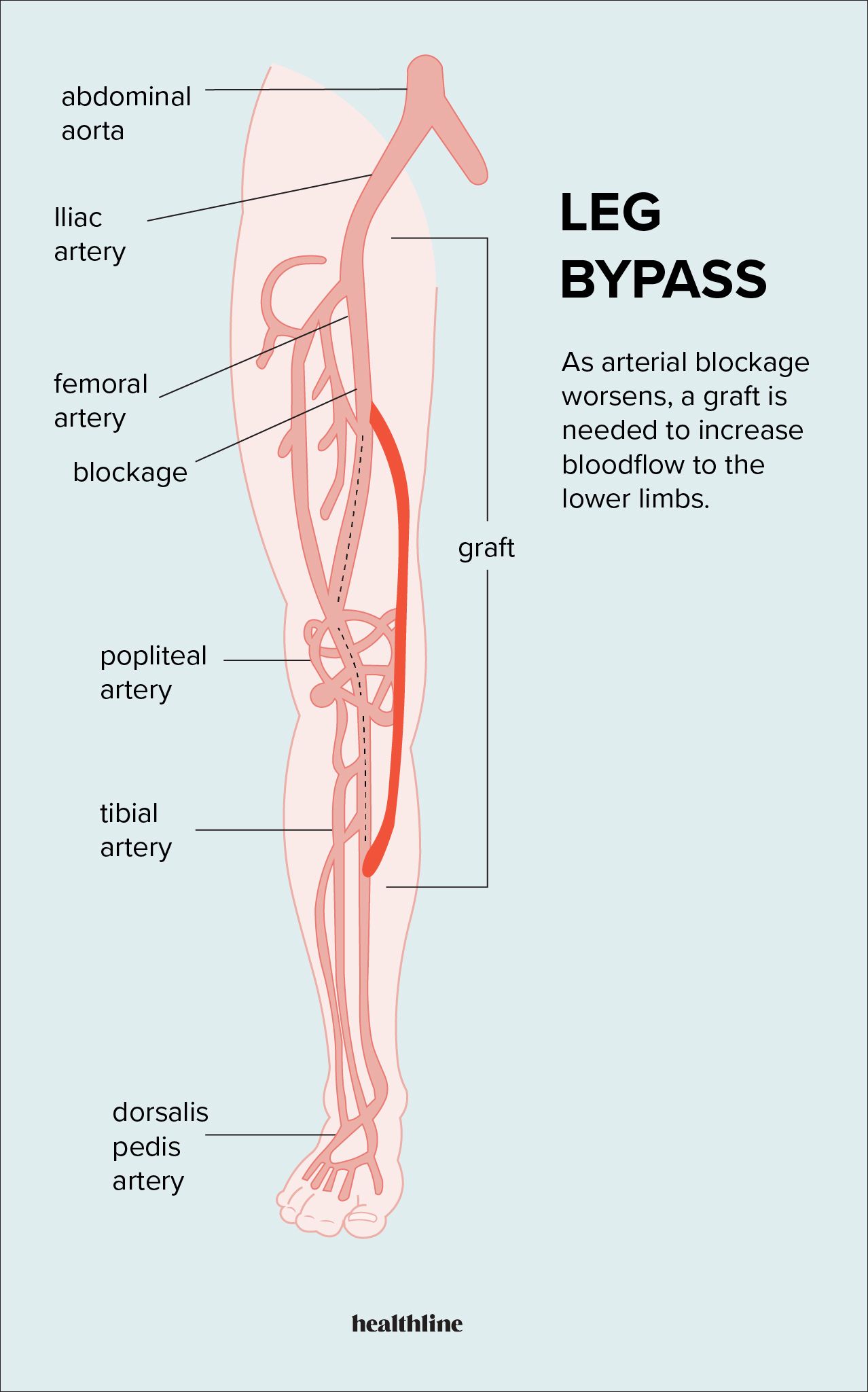The image is a detailed medical diagram of a leg bypass procedure. At the top left, it is titled "Leg Bypass," with a subheading that reads, "As arterial blockage worsens, a graft is needed to increase blood flow to the lower limbs." The main feature of the image is a depiction of a human leg, including all the major arteries labeled clearly from top to bottom: abdominal aorta, iliac artery, femoral artery, blockage, popliteal artery, tibial artery, and dorsalis pedis artery. The diagram highlights where the graft should be placed to alleviate the arterial blockage, with the existing arteries shown in a salmon color and the graft itself depicted in a brighter red. The background of the image is a light blue, and at the bottom center, the word "Healthline" is prominently displayed. The detailed labels and color distinctions help to illustrate the procedure effectively.